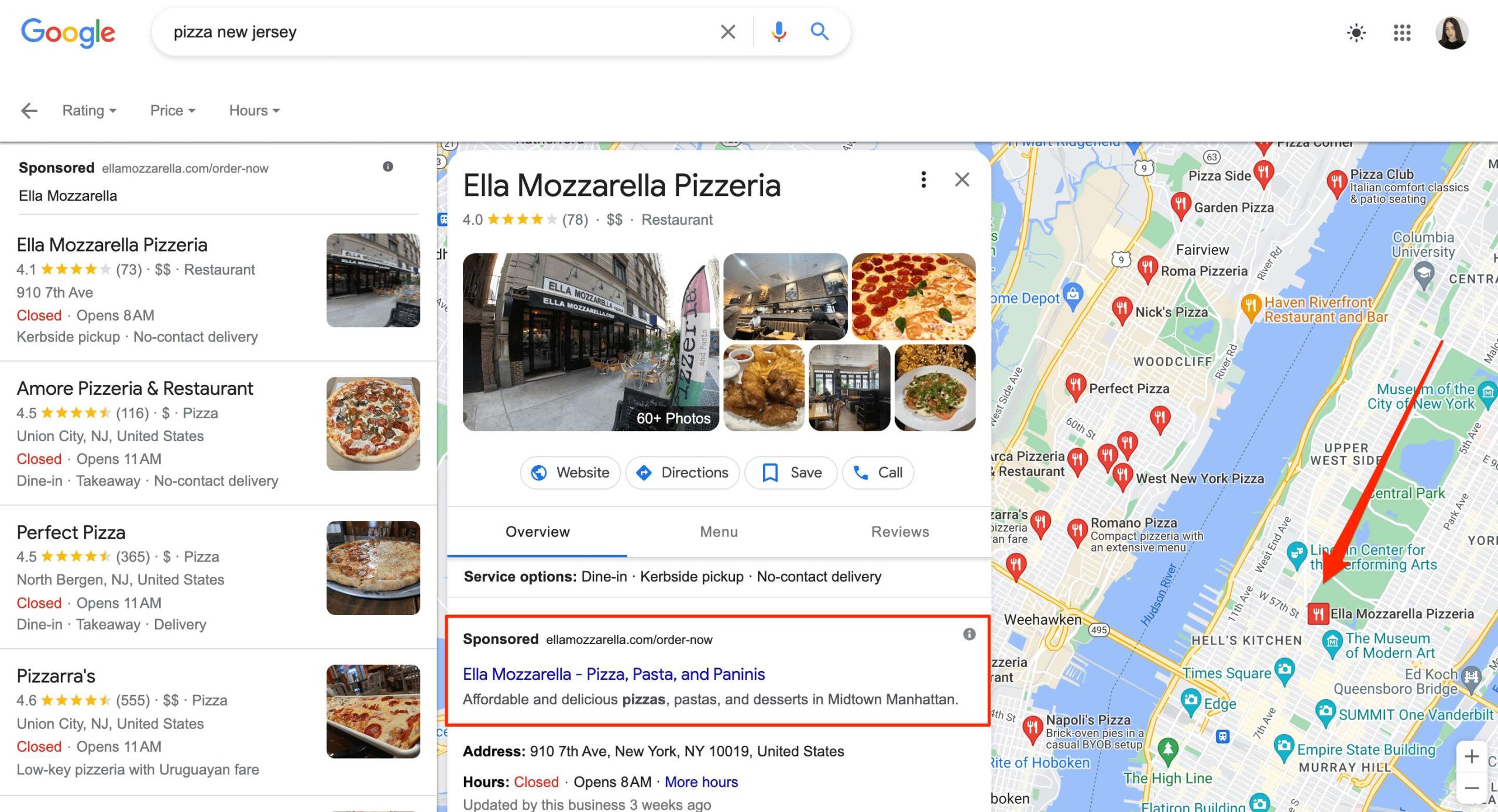In this Google Maps screenshot, a search for "Pizza New Jersey" is depicted at the top of the interface. The search results displayed are for various pizza restaurants in New Jersey. On the left side of the screen, there is a prominent sponsored link for Ella Mozzarella Pizzeria, highlighted with a red border. This pizzeria boasts a 4.1-star rating. Below it, several other pizza restaurants are listed, including Amore Pizzeria and Restaurant, which has a 4.5-star rating, Perfect Pizza also with a 4.5-star rating, and Pizzara's with a high rating of 4.6 stars. The selected search result, Ella Mozzarella Pizzeria, appears towards the center of the map on the right side. The map features various icons indicating the locations of these pizzerias around New Jersey, with a red arrow specifically pointing to the Ella Mozzarella Pizzeria icon, which is situated near the center.